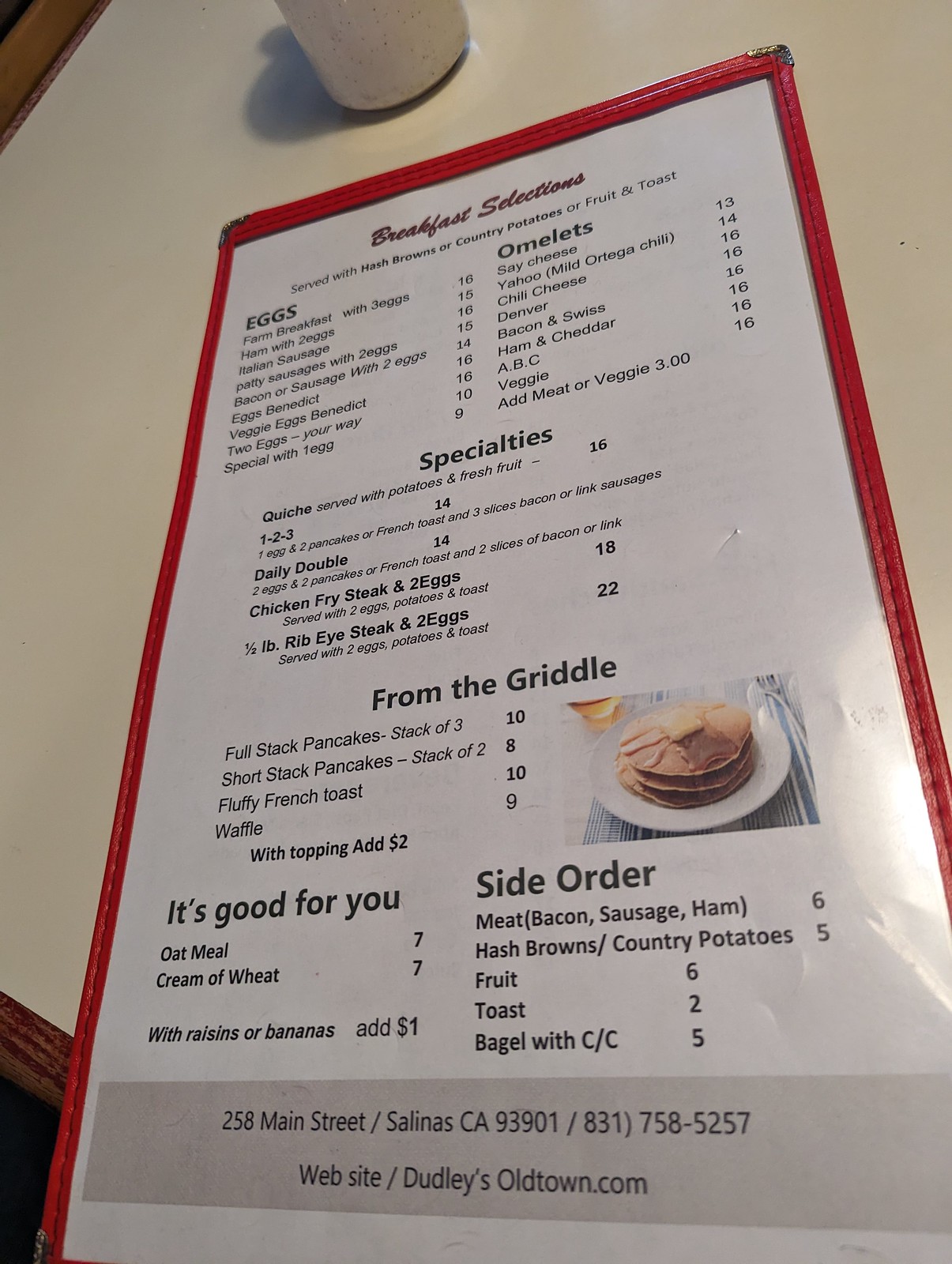The photograph captures a detailed view of a breakfast menu set on a white table from a slight angle, causing the bottom of the menu to appear closer than the top. The menu itself is characterized by a red outlined cover with a laminated white paper inside. The paper features vibrant images, notably of brown pancakes topped with butter on a white plate. A white coffee cup with dots is positioned above the menu in the background.

The menu header reads "Breakfast Selections," featuring various sections such as "Eggs," "Omelets," "Specialties," "From the Griddle," "It's Good for You," and "Side Orders." Detailed listings under these sections include:

- **Eggs:** Options range from a Farm Breakfast with three eggs ($16) to more specific combinations like Ham with two eggs ($15) and Eggs Benedict ($16).
  
- **Omelettes:** Choices include Cheese ($13), Denver ($16), and Ham and Cheddar ($16).

- **Specialties:** Items like Quiche served with potatoes and fresh fruit ($16) and a 1/2 Pound Ribeye Steak and two eggs ($22) are highlighted.

- **From the Griddle:** This section showcases the pictured pancakes, offering a Full Stack (three pancakes for $10) or Short Stack (two pancakes for $8). Additionally, it includes Fluffy French Toast ($10) and Waffles ($9) with optional toppings for an extra $2.

- **It's Good for You:** Features healthier options such as Oatmeal ($7) and Cream of Wheat ($7), with add-ins like raisins or bananas for $1.

- **Side Orders:** Includes Meat options like bacon, sausage, or ham ($6), Hash Browns or Country Potatoes ($5), Toast ($2), and Bagel with Cream Cheese ($5).

At the bottom of the menu, the address and contact information for the restaurant, Dudley's Old Town, is displayed: 258 Main Street, Salinas, California 93901, phone number 831-758-5257, and website DudleysOldTown.com.